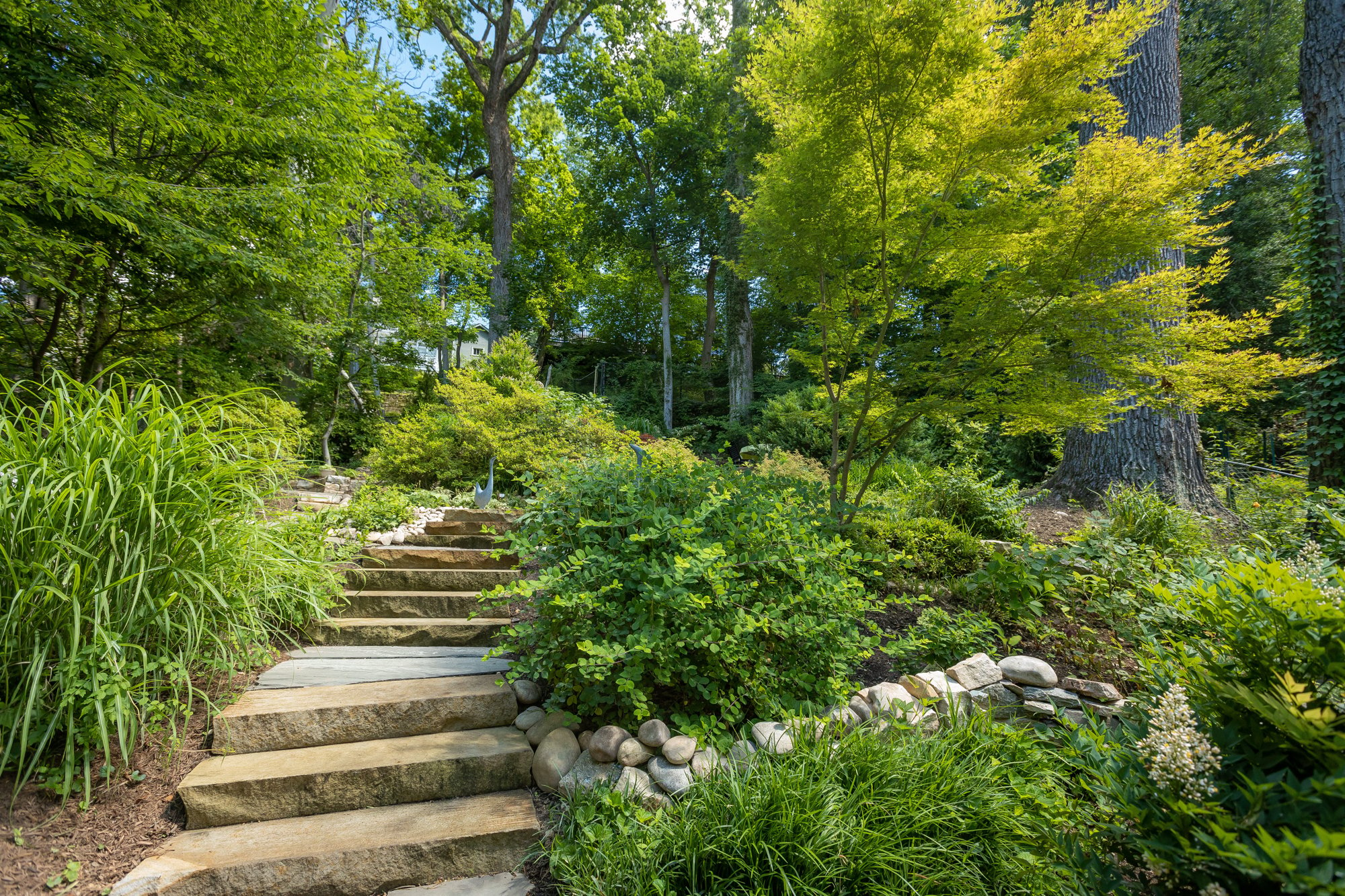An inviting outdoor photograph captures a lush, green natural area that appears to be a well-maintained botanical garden or a frequently visited forest. In the foreground, a row of stone steps ascends gently up a hill, interspersed with flat sections before continuing higher into the verdant landscape. The steps are flanked by very green bushes and bordered on both sides by smaller lush trees, with taller, mature trees towering in the background. A mix of white and flat rocks are dispersed around the area, contributing to the natural charm. About halfway up the steps, a row of rocks forms a retaining barrier for the soil, supporting various plants. The scene is complemented by wild grass sprouting at the base of the steps and a few wildflowers dotted around, while bare patches of soil peek through on the left side. Above, the blue sky peeks through the dense canopy of green, adding to the serene and picturesque atmosphere.